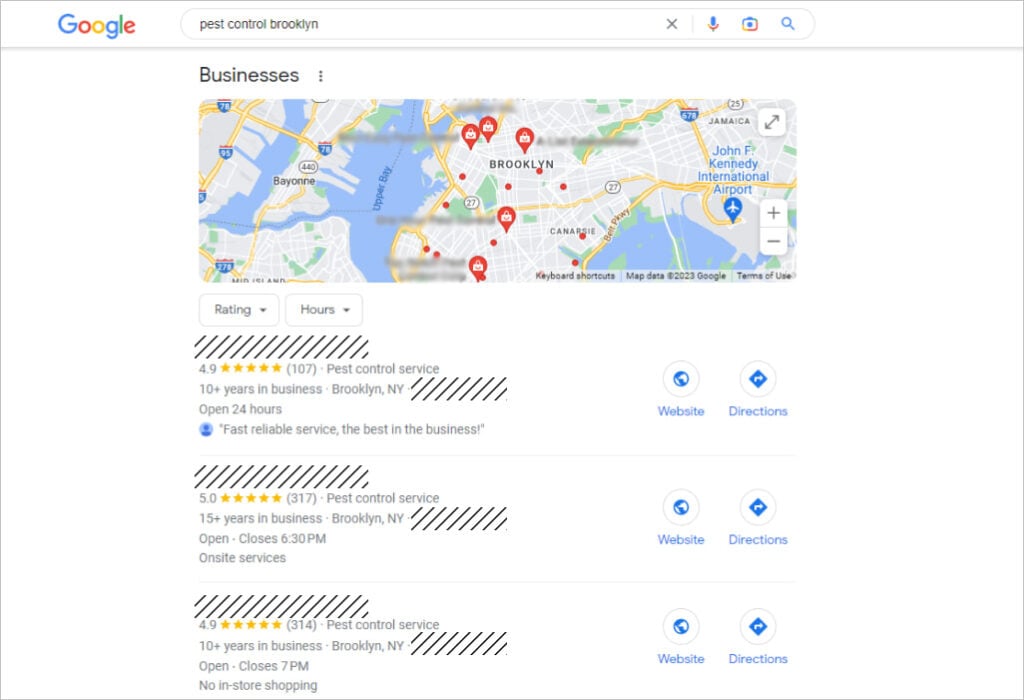This image shows a Google search results page for "pest control Brooklyn." In the upper left corner, the Google logo is prominently displayed. The search query itself, "pest control Brooklyn," is entered in the search bar. Below the search bar, there is a map of Brooklyn featuring blue areas to represent water and several locations marked by red pins, identified as pest control services.

The map clearly shows "Brooklyn" written on it. Alongside the map are several listings featuring pest control businesses. Each listing provides detailed information, some of which is struck through for privacy or naming reasons.

1. The first listing, marked with a white and gray diagonal stripe banner, has a rating of 4.9 stars with 107 reviews. It highlights "pest control services," mentions over 10 years in business, and states that the business is located in Brooklyn. Additional details include "open 24 hours," "fast, reliable service," and "the best in the business."

2. The second listing has a perfect 5-star rating based on 317 reviews. It indicates the business has been operational for over 15 years in Brooklyn, New York. Some details are struck through, but it mentions "open," "closes 6:30 p.m.," and "on-site service" as key features.

3. The third listing, again with its name struck through, holds a 4.9-star rating from 314 reviews. This business is described as offering pest control services for over 10 years in Brooklyn, New York. Despite some struck-through information, it highlights "open," "closes at 7 p.m.," and notes that there's "no in-store shopping."

All listings prominently display the "get directions" and "website" links for further user convenience.